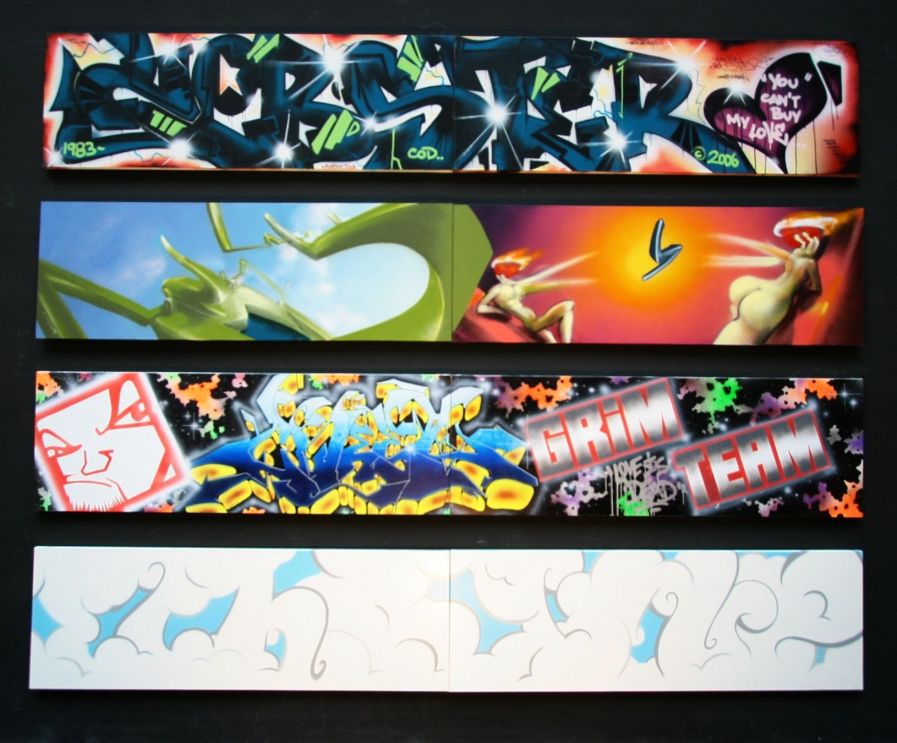The image features four vertically arranged, elongated rectangular frames set against a black background. Each frame showcases different styles and themes of artwork with black borders separating them.

- The top frame is a vibrant graffiti-style design with dark blue and black lettering on a red and white backdrop. Prominently displayed on the right is a fragmented heart with the words "You can't buy my love."
- The second frame showcases a split scene: on the left, a blue sky with what appears to be the green head and arms of a praying mantis. On the right, set against a red background, are two nude anime-style figures with flaming red hair, appearing to be mid-action.
- The third frame is an abstract composition with varied colors including yellow, blue, orange, green, and purple. A red, somewhat cartoony-looking face emerges from the left side, while the right side has the text "Grim Team" in silver letters against a red backdrop.
- The bottom frame is dominated by a light blue background interspersed with white areas that look like torn paper revealing the blue beneath, resembling a cloudy sky.

This eclectic mix of imagery combines elements of graffiti, abstract art, and anime, each contributing to the overall vibrant and diverse aesthetic.